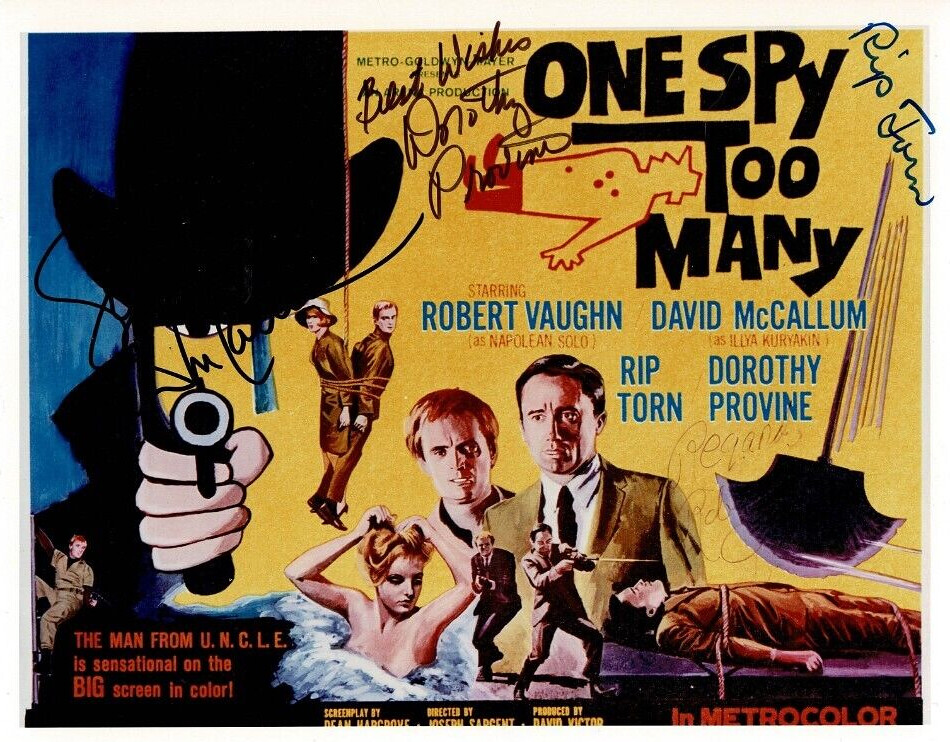This vintage movie poster for "One Spy Too Many" is richly detailed and appears hand-autographed with "Best Wishes, Dorothy Provine" along with Rip Torn's signature. The poster features an array of action-packed scenes including a gangster's hat-clad figure with a gun, a dynamic image of a man climbing a wall, and a bold statement declaring "The Man from U.N.C.L.E. is sensational on the big screen in color."

Prominent cast names like Robert Vaughn as Napoleon Solo, David McCallum as Illya Kuryakin, Rip Torn, and Dorothy Provine are displayed, though some text is faded. The left side showcases another autograph of an indiscernible name. The dramatic visuals include two men tied together dangling from a rope, five individuals facing the viewer, a man tied to a table beneath a swinging guillotine blade, and elements like a cartoonish dead body. The chaotic and thrilling essence of the film is encapsulated in this evocative poster, making it a collector's gem.